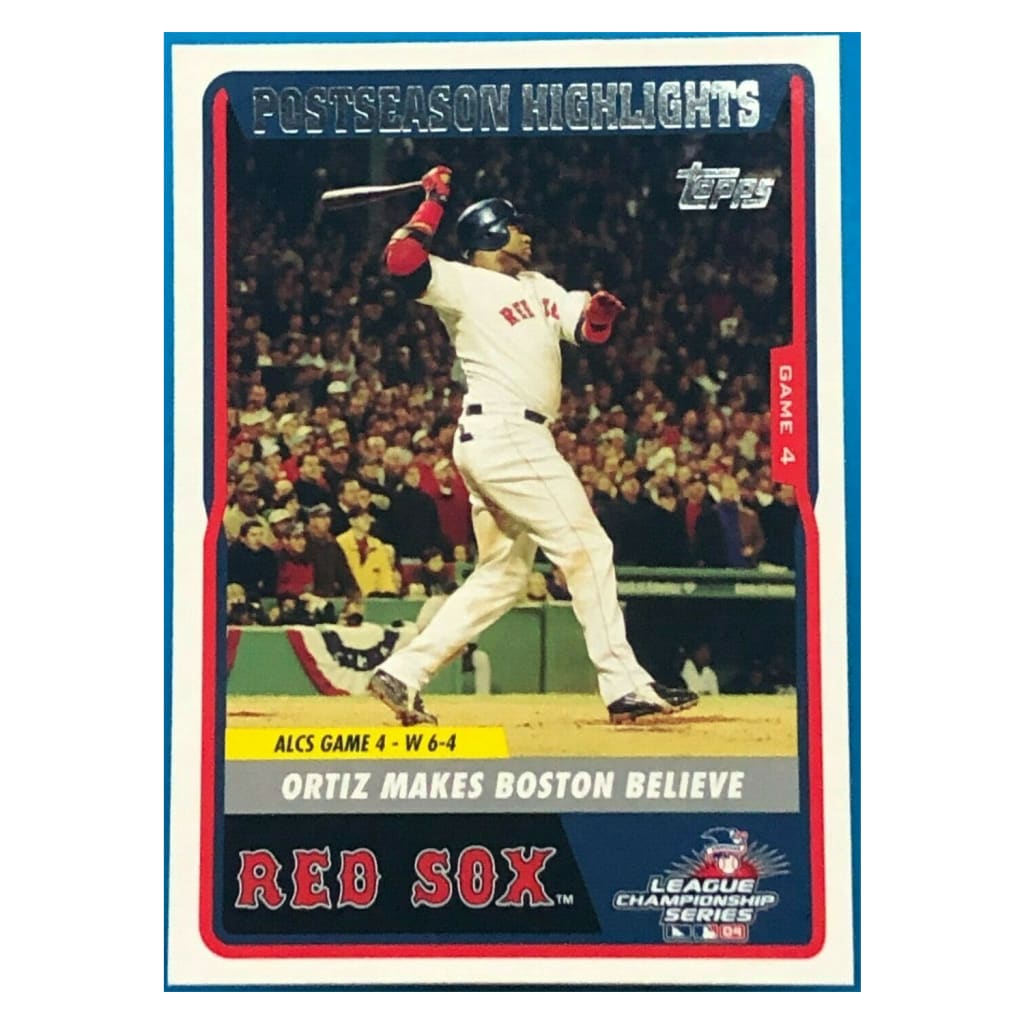This is a detailed baseball card featuring Ortiz, a player from the Boston Red Sox, commemorating a pivotal moment in ALCS Game 4 with a 6-4 victory. The card proudly highlights the caption "Ortiz makes Boston believe," symbolizing his significant impact on the game. The top of the card reads "Post-Season Highlights" in silver, with the company name, Tops, in the upper right corner. The main image captures Ortiz mid-swing, having just hit the ball, with fans and American flags visible in the background. The card prominently displays "Game 4" on the right side and includes the Red Sox logo in the bottom left corner, along with a blue and red League Championship Series logo in the bottom right. Encased in white and blue borders, the card's design hints at its vintage nature, even though it does not specify the year. This standard baseball card is a tribute to a memorable moment in baseball history.